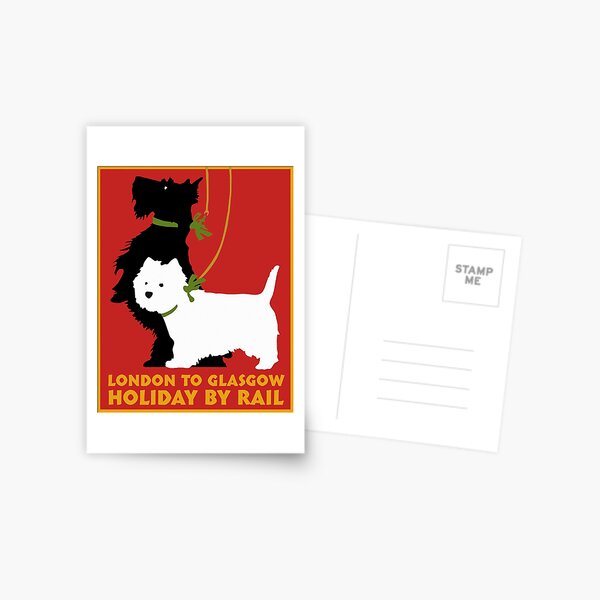This image showcases both the front and back of a postcard. The front features a vertical, cartoon-like illustration of two dogs against a white background. Central to the design is a red box outlined in yellow. The box contains the black silhouette of a dog standing on its hind legs to the left, and a white dog standing on all fours, both wearing green collars with bows. The text within the red box, written in yellow, reads: "London to Glasgow, holiday by rail." Below this is the back of the postcard, displayed in a landscape orientation with a light grey background, featuring the typical blackish light-blue lines for an address and a designated area for a stamp labeled "stamp me."